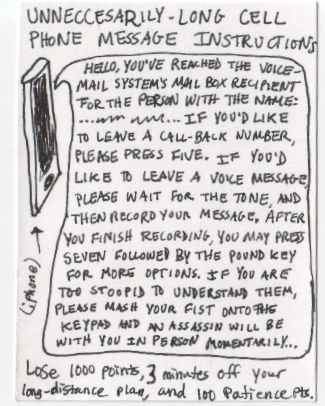The image depicts a detailed sketch featuring a smartphone turned on its side, viewed from an angled perspective on the left.  The drawing includes a handwritten note that reads "unnecessarily long cell phone message instructions." The primary focus is a large comic-style speech bubble containing a sarcastic and verbose voicemail message. The message humorously states:

"Hello, you've reached the voicemail system mailbox recipient for the person with the name blah blah blah. If you'd like to leave a callback number, please press 5. If you would like to leave a voice message, please wait for the tone and then record your message. After you finish recording, you may press 7, followed by the pound key for more options. If you are too stupid (spelled s-t-o-o-p-i-d) to understand them, please smash your fist onto the keypad and an assassin will be with you in person momentarily."

Beneath this message, there is a note indicating penalties: "lose 1,000 points, three minutes off your long-distance plan, and 100 patient points."